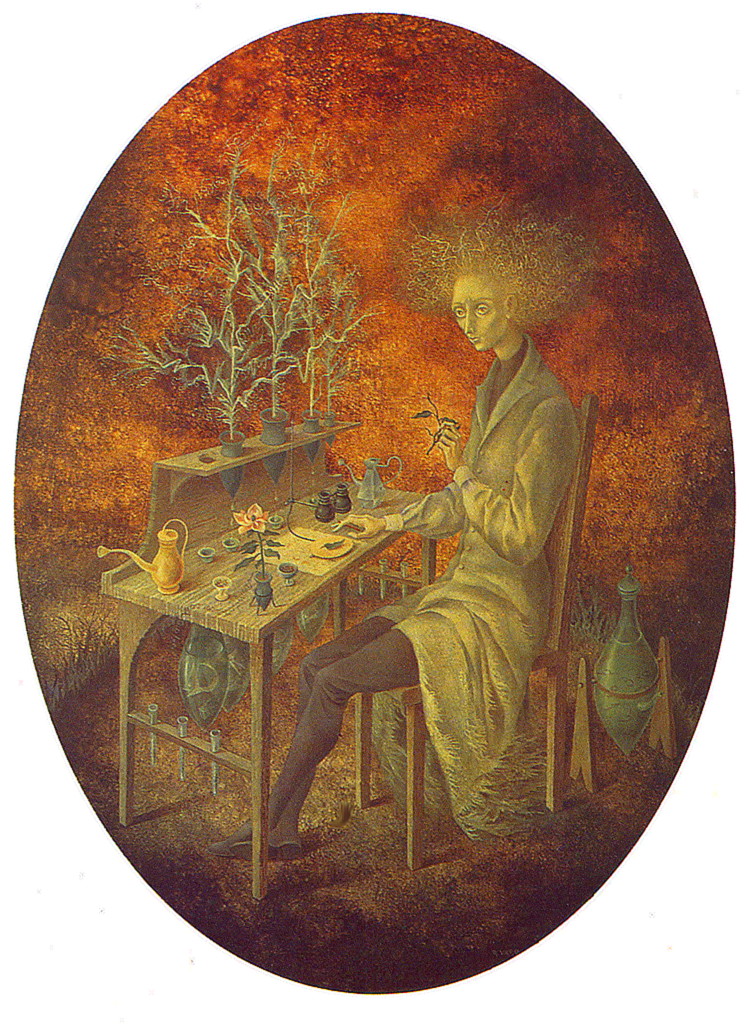The image depicts a gaunt woman seated at a wooden desk adorned with botanical elements, suggesting a deep interest in plants. Her hair is chaotic and wild, reminiscent of Albert Einstein’s iconic look, and even takes on a twig-like appearance, enhancing the overall disheveled aesthetic. She wears a light green overcoat that flows like a dress and dark brown pants, with her yellowish skin adding to the unique appearance. 

Before her, the desk is organized with various plant-related items including circular plant holders with budding tree branches and other floral decorations. A small watering can and several vases are also present, reinforcing the botanical theme. Her left hand holds a leaf, hinting at a botanical experiment or study.

The background sets off the scene with an amber-orange, fiery brown hue, adding depth and a somewhat otherworldly ambiance to the setting. The image is egg-shaped, featuring a range of colors such as yellow, green, pink, brown, orange, black, white, gray, and tan, creating a vivid and detailed portrayal of the woman and her botanical environment.